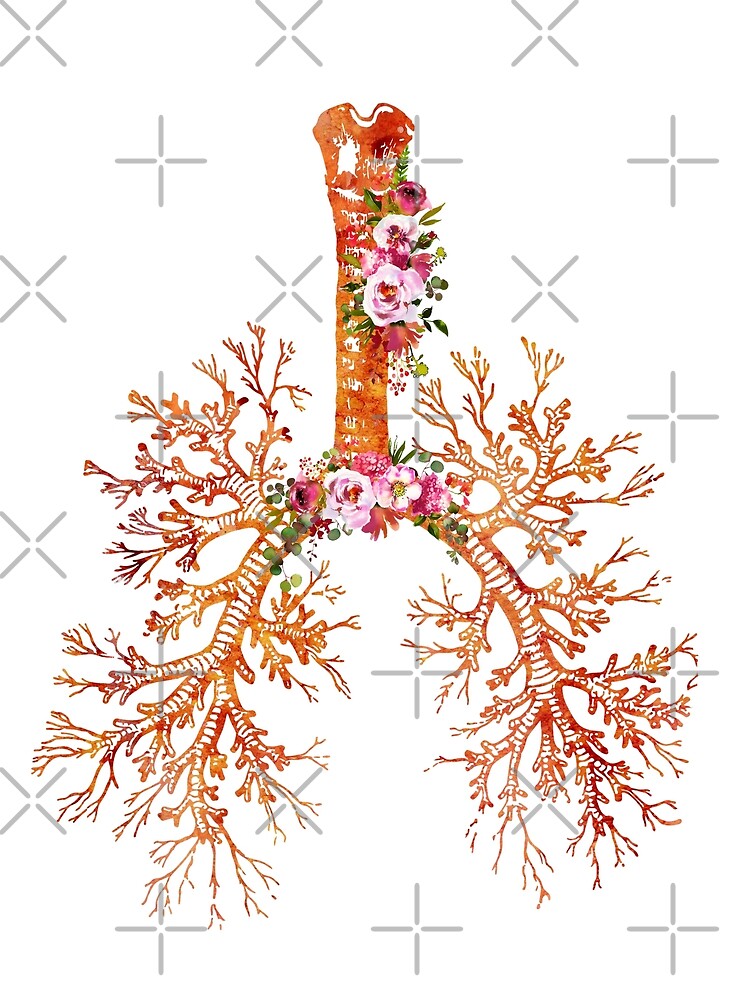This artistic painting features an abstract representation of the lungs and bronchial tubes, visually resembling a branching network of roots or a flower stem. Set against a fully white background, the central structure is a brown tube that bifurcates, simulating the intricate network of bronchial paths. The tubes are brown with ribbed white designs, giving them a textured, organic feel. Warm hues of red, orange, and yellow blend into the lines, enhancing the naturalistic warmth of the image. Various capillaries branch outwards, mimicking the detailed anatomy of the respiratory system.

Adding a touch of vibrancy, clusters of wild roses in shades of pink, light pink, dark pink, and violet, along with green leaves, adorn the artwork. These flowers are prominently placed at the top of the trunk and at key branching points, adding a splash of color and life to the otherwise anatomical structure. The juxtaposition of botanical elements with anatomical structures results in a visually striking and thought-provoking piece.